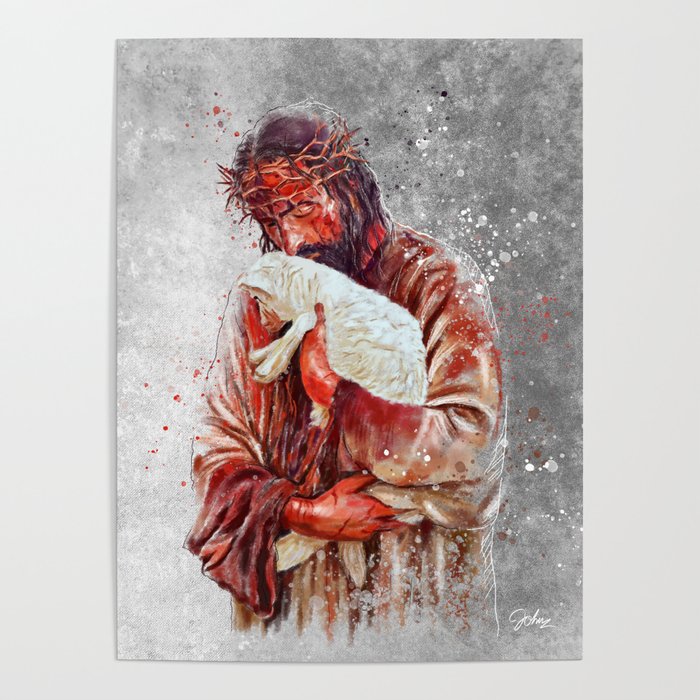The image is a detailed painting of Jesus Christ set against a gray, white, and blackish charcoal background, hanging on a gray wall. Jesus is depicted with a crown of thorns on his head, causing blood to stream down his face, onto his long brown hair, brown mustache, and beard. He is wearing a long, white robe that is heavily stained with blood. His eyes are closed, and he is gently holding a small white lamb close to his face, nuzzling it with his eyes shut as if in a protective embrace. The lamb has a slight blood mark near its mouth, possibly from Jesus’ hand, but remains largely unsoiled. The hands of Jesus are visibly dripping with blood, and the background contains scattered blood splatters. The painting is signed by the artist in the bottom right-hand corner, though the name "John" is somewhat hard to decipher amidst the vivid and haunting details.